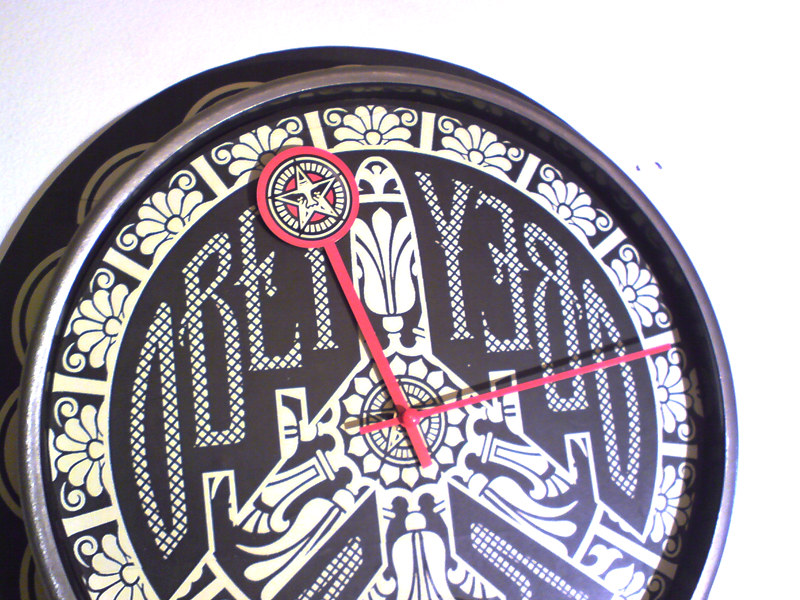This close-up image captures three-fourths of a uniquely designed clock against a plain white background, with the very bottom portion of the clock obscured. The clock's frame is edged in sleek silver metal, adding a modern touch to its appearance. The clock face features an artistic depiction of what seems to be three-fourths of a sunflower, entirely rendered in white. Within this floral design, eleven distinct petals are visible.

At the heart of the clock lies an intricate illustration of an airplane adorned with white patterns. This airplane features decorative tassels and a centerpiece that combines a floral motif with a star at its core. The background of the clock's face is a solid brown hue, creating a striking contrast with the white designs. Flanking the airplane on both sides are the words "OBEY" – correctly oriented on the left and mirrored as "YEBO" on the right.

The clock's hands are painted in a vivid red, adding a splash of color to the monochromatic face. One of the clock hands is uniquely designed with a circular emblem that includes a star, resembling a face within it. This blend of contemporary elements and detailed artistry makes the clock a fascinating piece to behold.